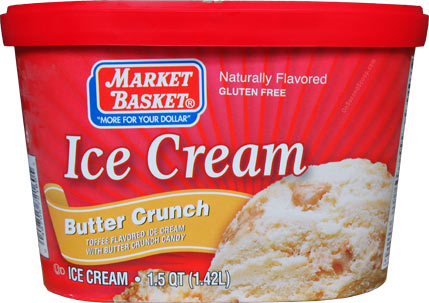This image depicts a 1.5-quart (1.42 liters) container of Market Basket ice cream, prominently featuring a red theme. Both the top and the lid are red, while the container itself is a lighter shade of red. The brand name, "Market Basket," is displayed along with its slogan, "More for Your Dollar." The ice cream is naturally flavored and gluten-free, as indicated in white font. The flavor, Butter Crunch, is highlighted on a yellow ribbon that traverses the container, describing the contents as "toffee flavored ice cream with butter crunch candy." A scoop of the ice cream is shown on the right side of the container, portraying a creamy white color with golden brown flecks of toffee. The background sports a design reminiscent of sun rays emanating into the red. Additionally, the nutritional information and SKU number are partially visible on the edges of the container.